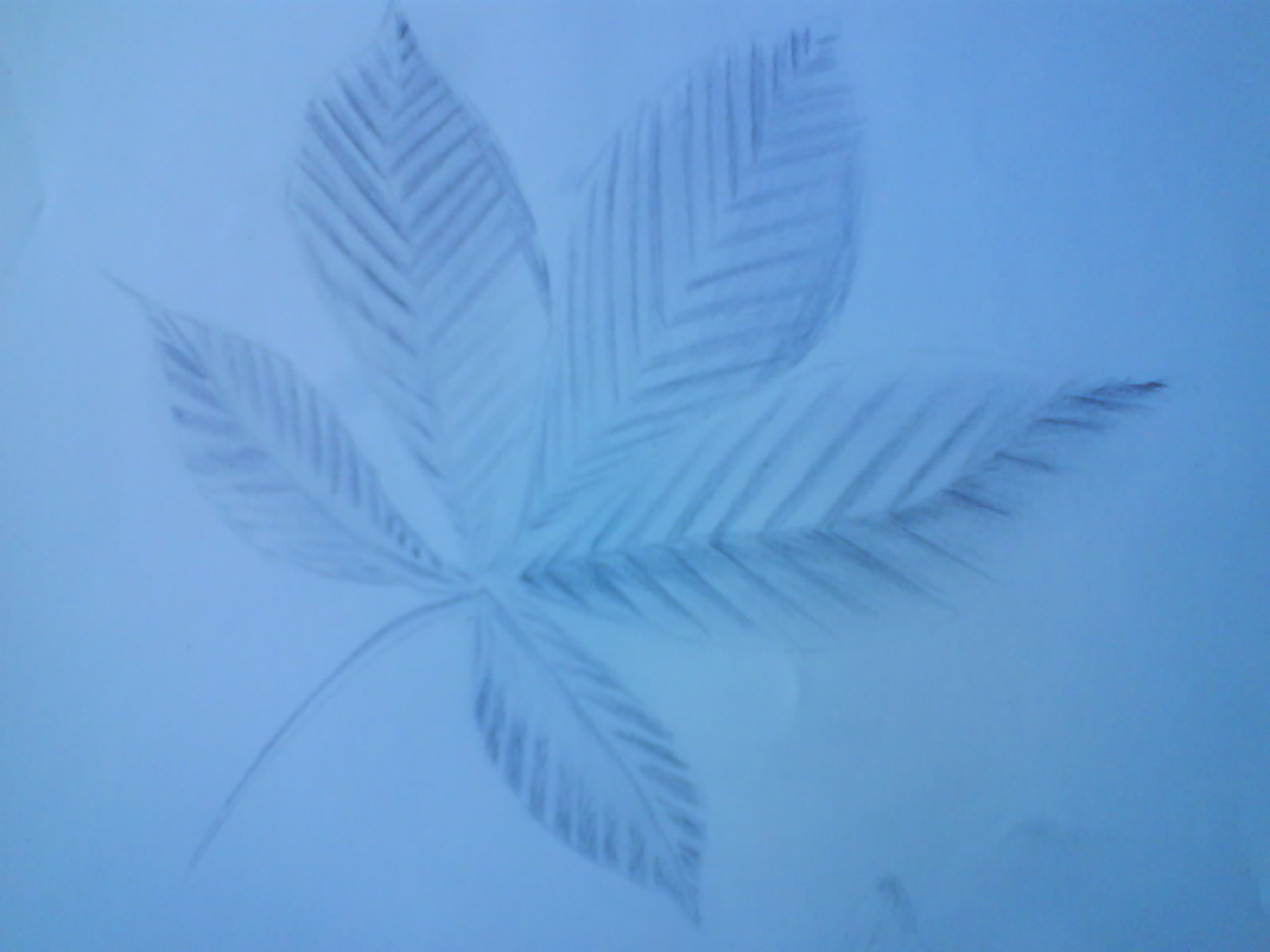The image is a photograph of a drawing or sketch with a distinct blue tint, either due to lighting conditions or the color of the paper itself. The drawing depicts a plant with five long, thin leaves attached to a single stem, arranged in a fan-like spread. Each leaf features detailed shading and numerous diagonal lines indicating the ribbing or veins, created with dark blue or charcoal strokes. The leaf design takes up approximately 80% of the image, emphasizing its prominence against the minimalistic light blue background. The image contains no additional elements, such as writing, people, animals, buildings, mechanical objects, signs, or vehicles.